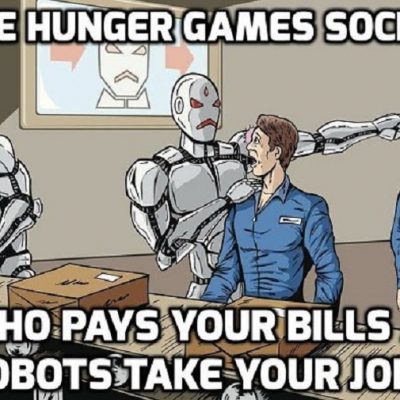The image appears to be a screen grab from a comic cartoon, depicting a dramatic scene. In the foreground, there is a white robot with a mechanical appearance featuring red eyes and a red mouth, giving it an ominous and intense expression. The robot is positioned behind a brown-haired, light-skinned man who is dressed in a blue shirt with a button-up collar and a white name tag. The robot's right hand is placed on the man's right shoulder while its left hand points outward to the right. 

To the left of the frame, a partial view of another white robot's arm is visible, suggesting it shares a similar design. The background includes a tan wall, a dark beige floor, and a screen showing a close-up of a robot face with red arrows alongside, implying it's observing the characters. In front of the man, a table holds several brown wrapped packages. The image features white text that is partially cut off at the top and bottom: the top reads "eHungerGamesSoc" and the bottom is partially legible, displaying "Ho Pays Your Bills" with a subsequent line that seems to spell out "Bots Take Your Job."